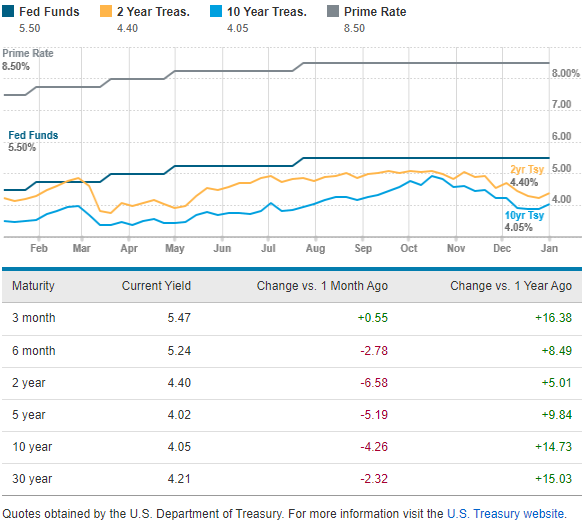In the top left corner, the red box reads "Fed Funds - 5.50%," and an orange box signifies the "Two-year Treasury - 4.40%." Adjacent to it, a blue square indicates the "10-year Treasury - 4.05%." A prominent gray square marks the "Primary - 8.50%," followed by another label "Primary - 8.5%," and "Dragon Lions, 8%." 

In the center, it lists "Fed Funds - 5.50%," and mentions "Two Lions" followed by "Dragon Lions, 10%." A yellow box represents the "Two-year Treasury - 4.0%," and a blue line indicates the "10-year Treasury - 4.05%." 

The timeline across the image spans from February to January, labeled sequentially: February, March, April, May, June, July, August, September, October, November, December, January. 

A gray rectangle contains maturity dates - "3.612-year," "5-year," "10-year," and "30-year" - and current yields: "5.57%," "5.204%," "4.40%," "4.02%," "4.05%," and "4.21%." This section also includes a comparison of the change in yields versus a month ago and versus a year ago:
- Change versus a month ago: +0.55, -2.78, -6.58, -4.19, -4.26, -2.32
- Change versus a year ago: +16.38, +8.49, +5.01, +9.84, +14.73, +15.03

Beneath this data, there's a disclaimer noting, "Quotes obtained by the U.S. Department of Treasury. For more information, visit the U.S. Treasury website." This section indicates a diverse range of U.S. Treasury information.